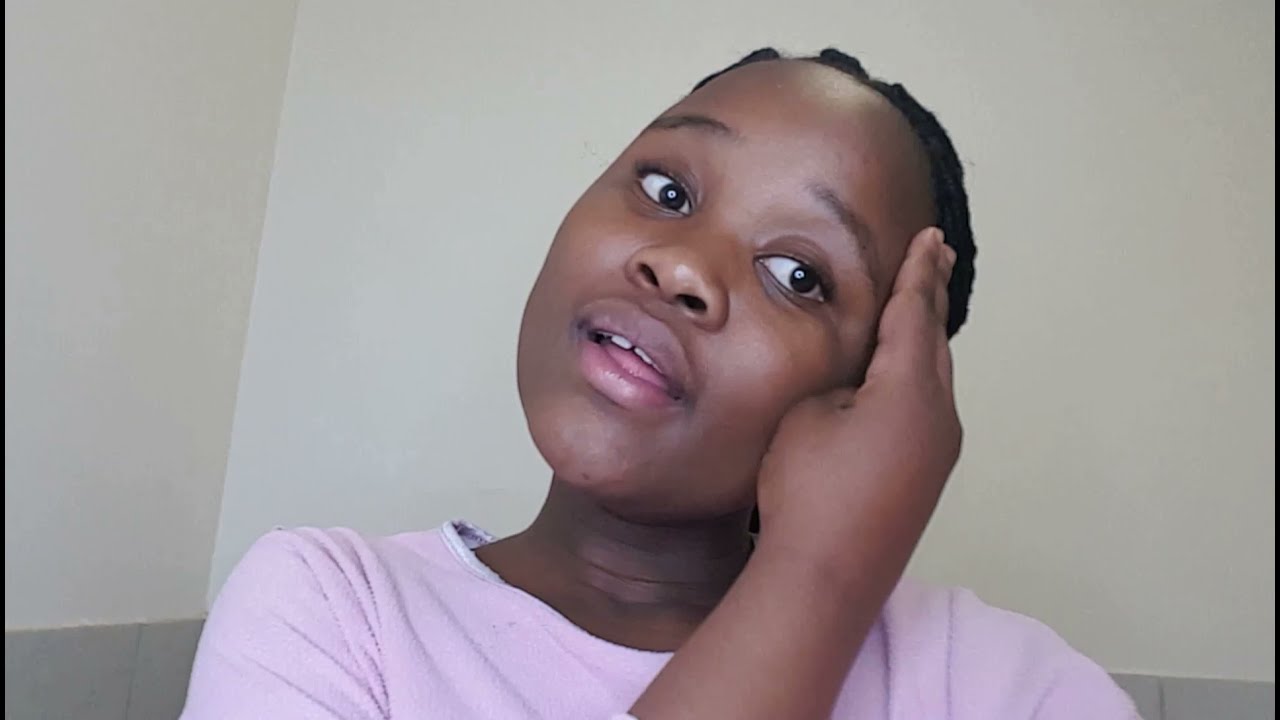The image is a detailed, expressive photograph of a young African-American girl with rich brown skin and dark, curly hair pulled back. She faces forward with her head slightly tilted to the right while using her right hand to touch the right side of her forehead, causing her arm to cross over her chest. She wears a light pink shirt and has a neutral facial expression. Her eyes are open and she looks slightly downward, her mouth slightly open, revealing her top front teeth and a hint of her pink tongue. The background features a pale yellow or cream-colored wall transitioning to a gray section at the bottom, possibly with a brick pattern.